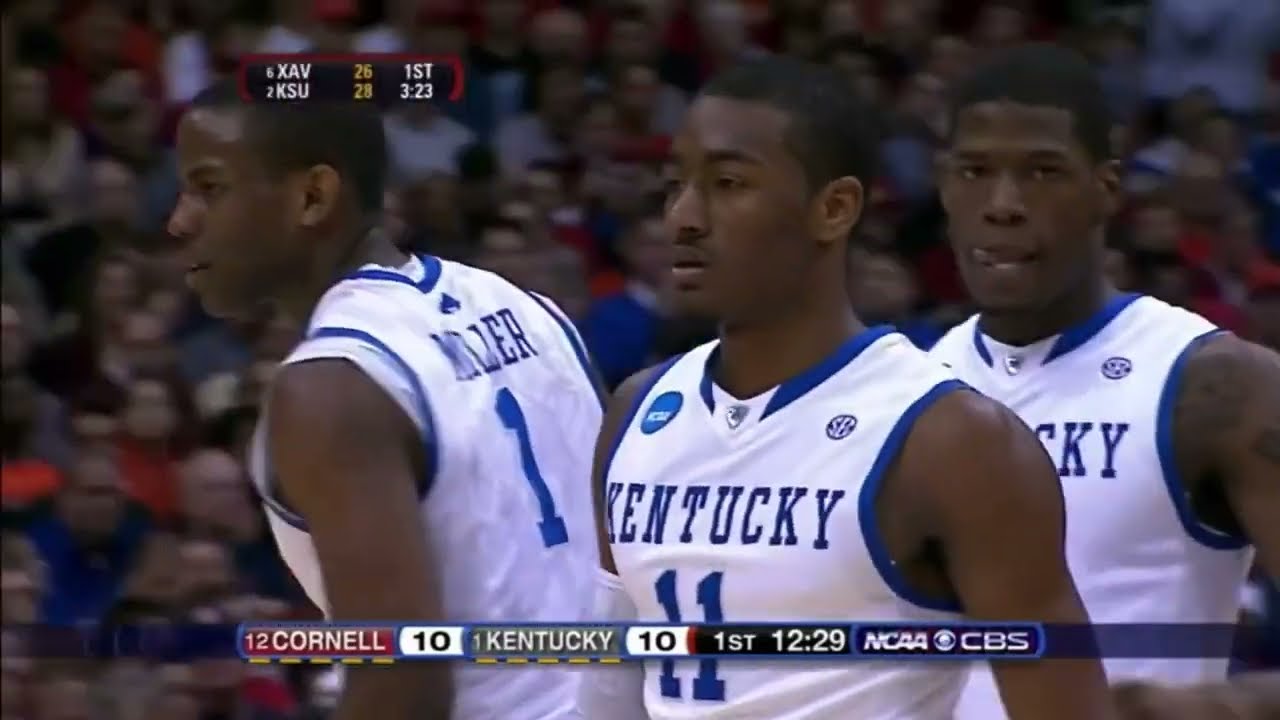The image is a still from a broadcast of a college basketball game featuring three Kentucky players against Cornell. At the center, John Wall is prominently displayed in a white Kentucky jersey with blue highlights, bearing the number 11. To his left is Miller, wearing the number one jersey and facing away from the camera. Another player stands to the right, with his hands on his hips, his tongue visible as he licks his lips. All three players are black men with short hair. The scoreboard at the bottom shows the game tied at 10-10 with 12:29 remaining in the first half, indicative of an NCAA match being aired on CBS, as mentioned in the lower right. Another score in the top left corner reveals a concurrent game between Xavier and Kansas State, with Kansas State leading 28-26 and 3:23 left in the first half. The background shows a blurred crowd, focusing the attention on the foreground players and game details.